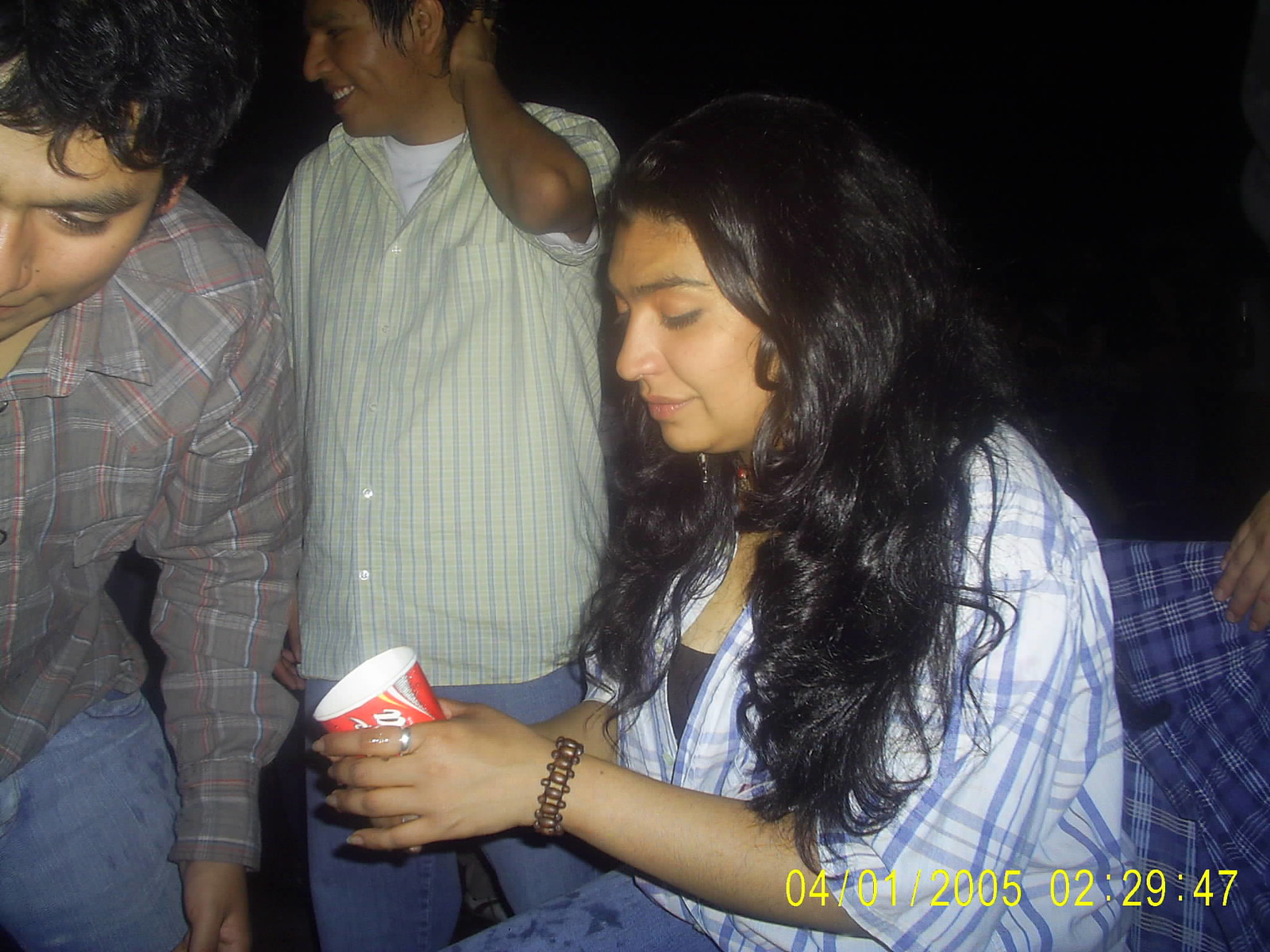In this image, the primary focus is a girl with long, curly black hair cascading down to her elbows. She wears a light blue and white plaid shirt over a black camisole and holds a red Coca-Cola cup while looking down at it, captured in her side profile. A silver ring adorns her index finger, and a brown bracelet circles her wrist. Flanking her are two men, neither of whom are looking at the camera. The man closest to her, wearing a yellow button-down shirt, has his hand resting on his neck and looks off to the side with a smile, while the other man in a brown and red plaid shirt gazes down at the floor. All three are wearing blue jeans. The background is completely black, suggesting it might be nighttime. In the bottom right of the image, there is a date and time stamp: April 1, 2005, at 02:29:47.